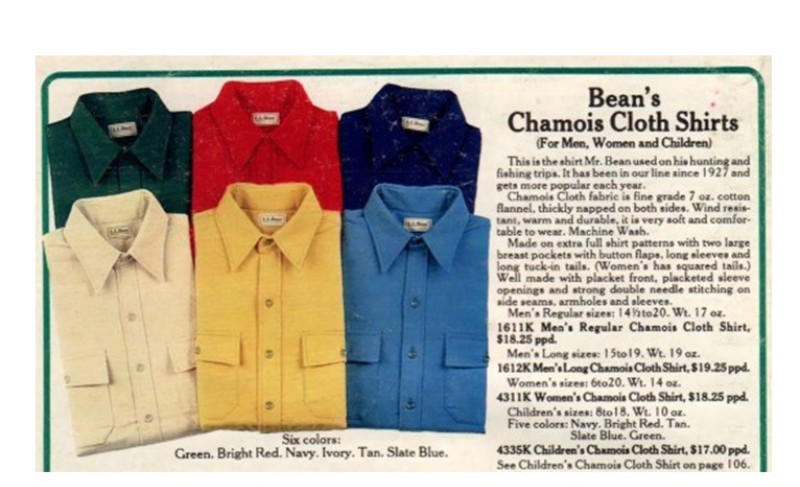This image displays a page from an L.L. Bean catalog, showcasing their Beans Chamois Cloth Shirts for men, women, and children. The 8 by 11 ad, set against a tan parchment-colored background, features black text headings and detailed descriptions of the shirts, including their prices, sizes, and styles. A green border frames the entire page. On the left two-thirds of the ad are images of six neatly-folded, long-sleeve collared shirts with two breast pockets each, arranged in two rows of three. The top row comprises shirts in forest green, bright red, and dark navy blue, while the bottom row includes shirts in beige, mustard yellow, and light blue. Beneath the shirts, the color names are listed in black text: green, bright red, navy, ivory, tan, and slate blue. The right side of the ad contains a comprehensive description of the shirts, emphasizing their enduring popularity since 1927, their durable 7-ounce cotton flannel fabric, and features such as wind resistance, softness, and machine washability. Additional details include design specifics like double pocket flaps, long tuck-in tails for men, and square tails for women, along with strong double-needle stitching on side seams, armholes, and sleeves. Pricing is detailed with men’s shirts at $18.25, longer versions at $19.25, women’s shirts also at $18.25, and children’s shirts at $17.